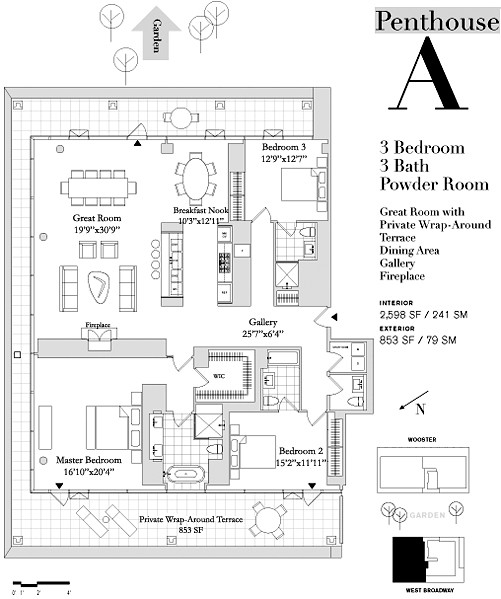This detailed floor plan provides an overhead view of a penthouse layout, depicted in a simplified blueprint style. At the top of the layout, a stout gray arrow marked "Garden" in black indicates the direction toward the garden area, which features four symbolically represented trees, each designed with a circular shape, a twig-like branch, and a trunk. 

The actual floor plan is outlined by a thin black border for interior walls and a stouter gray border for exterior walls. A scale in the bottom left corner, although illegible in terms of specific measurements, provides a reference for distinguishing spatial dimensions within the floor plan.

Central to the layout is a great room, which exhibits an open floor plan incorporating multiple functional areas. This room features a dining table with ten chairs, a breakfast nook with an oval table and six chairs, as well as a galley-style kitchen. Adjacent to these areas is a cozy fireplace accompanied by a seating area with a boomerang-shaped coffee table.

Behind the kitchen on the right side of the layout, Bedroom 3 is detailed with its dimensions, including an illustrated bed complete with two pillows, nightstands on either side, and even the edge of the sheets pulled down. An interior door from this bedroom swings open into a bathroom, which contains a commode, sink, and what appears to be a combined shower/tub. This bathroom also has a door leading to a hallway behind the kitchen.

Adjacent to this hallway is a gallery area, marked with its own dimensions, and an exterior door leading outside. Another door from the hallway provides access to a WC, though the exact function of this space remains unclear. 

The master bedroom, located in the layout, includes a two-sink vanity, a tub (possibly a soaker tub), a separate shower, and a toilet. Additionally, Bedroom 2 and its dimensions are noted.

The plan also highlights a private wraparound terrace, complete with an exterior table and four chairs, as well as two chaise lounges, offering an inviting outdoor space.

Across the right side of the image, large text reads "Penthouse A," describing the overall unit as comprising three bedrooms, three bathrooms, a powder room, a great room with private wraparound terrace, a dining area, gallery, and fireplace. The interior spans 2,598 square feet (241 square meters), while the exterior measures 853 square feet (79 square meters).

A directional arrow indicates north as being to the bottom left (southwest). Below this, a schematic labeled "Rooster" (possibly a potting shed) and references to a garden and West Broadway, which could signify the street fronting the property, complete the detailed floor plan.